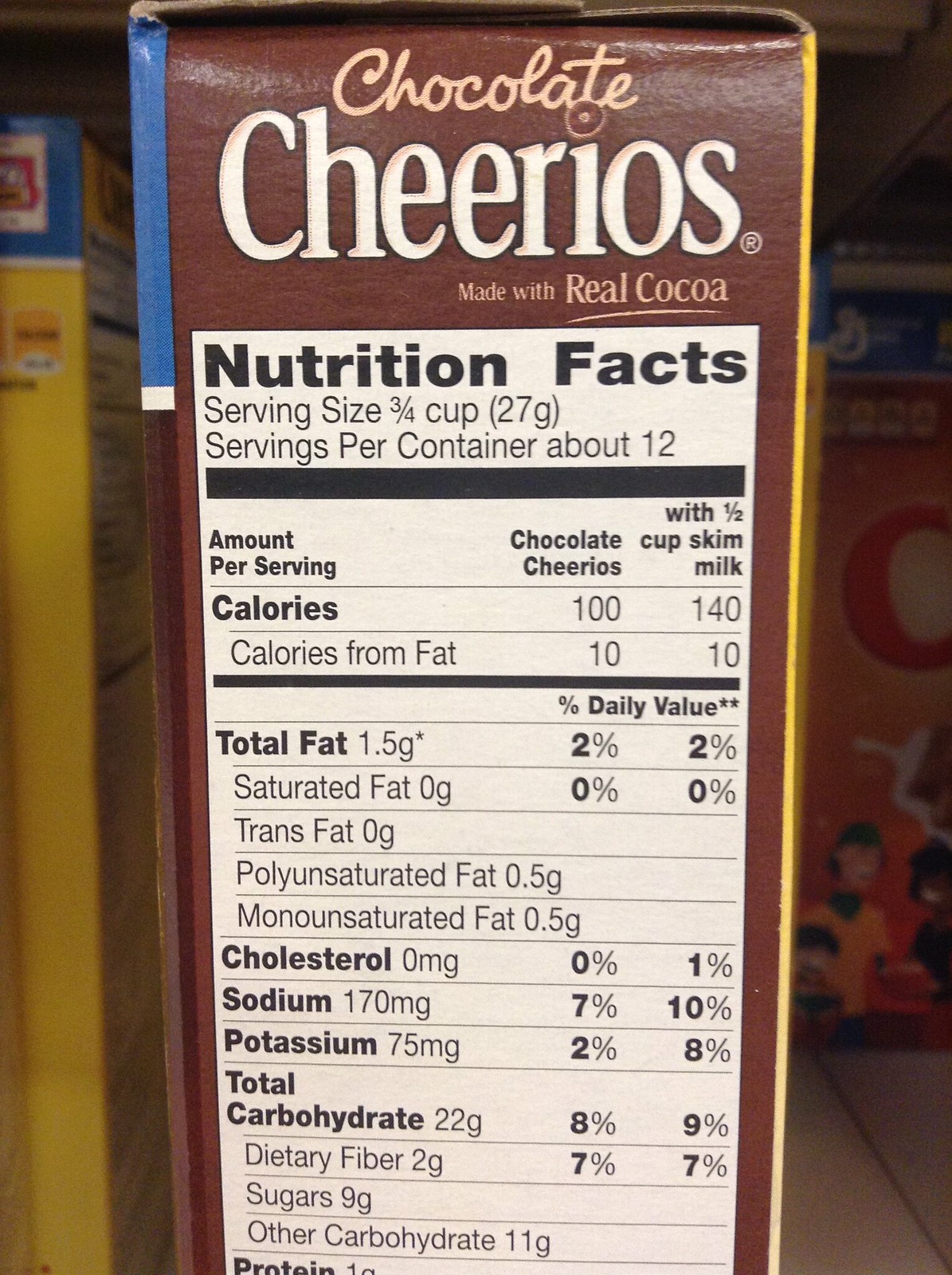The image depicts a close-up, first-person perspective of the side of a brown cereal box in a supermarket, specifically focusing on the nutritional facts and branding details. At the top of the box, in cursive beige lettering, it says "chocolate," followed by "Cheerios" in bold white text. Underneath, in smaller beige text, it states "made with real cocoa." The nutrition facts label dominates the middle part of the image, detailing serving sizes, caloric content, and various nutritional values such as total fats, sodium, and carbohydrates. The label reads: Serving size 3/4 cup (27 grams), servings per container about 12, calories per serving 100, and other detailed breakdowns of fats, cholesterol, sodium, and more. Both sides of the image show portions of adjacent cereal boxes, with a yellow box on the left and an orange box on the right, where part of a red letter "C" is visible. The detailed nutrition facts include: total fat 1.5 grams (2% daily value), saturated fat 0 grams, trans fat 0 grams, polyunsaturated fat 0.5 grams, monounsaturated fat 0.5 grams, cholesterol 0 milligrams (0% daily value), sodium 170 milligrams, potassium 75 milligrams, total carbohydrates 22 grams (8% daily value), dietary fiber 2 grams (7% daily value), sugars 9 grams, and other carbohydrates 11 grams. The remainder of the label is cut off at the bottom.